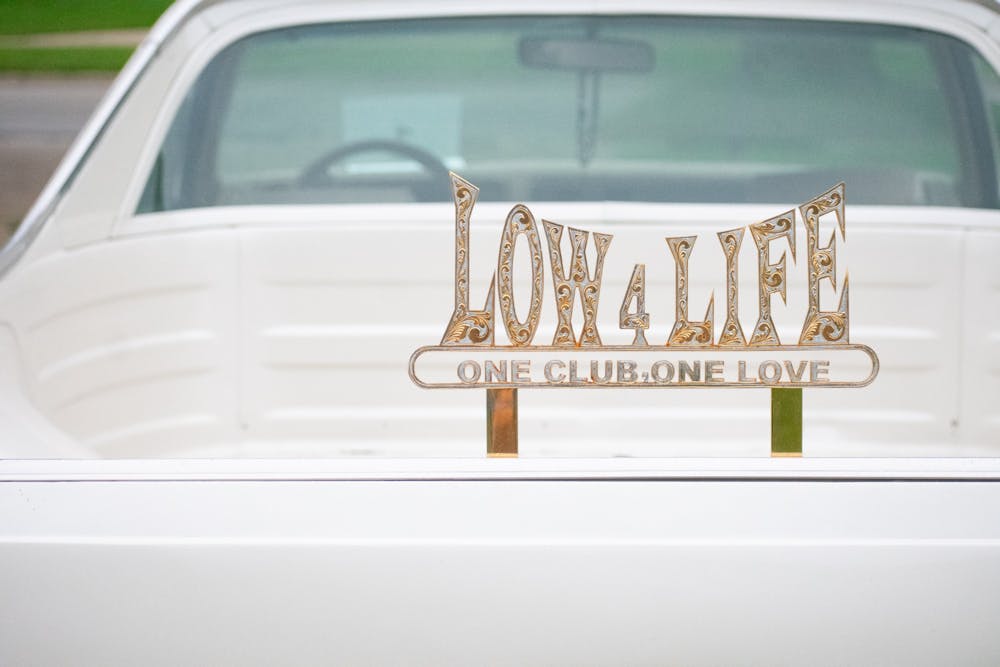The image depicts the rear of a white El Camino, a vehicle that resembles a subcompact-sized pickup truck. Visible in the frame are the rear wheel and the rearview mirror inside the cabin, from which a chain or rosary bead dangles. Prominently, there is an ornamental sign affixed to the lowered tailgate of the truck. The sign, featuring a metallic finish that appears to be either brass or tin-plated, bears the inscription "Low 4 Life" in large, gold-bordered letters with the number '4' between "Low" and "Life." Below this, in a rounded rectangle, the phrase "One Club, One Love" is elegantly displayed in silver. The sign is supported by two posts, with one post being copper-colored and the other green.